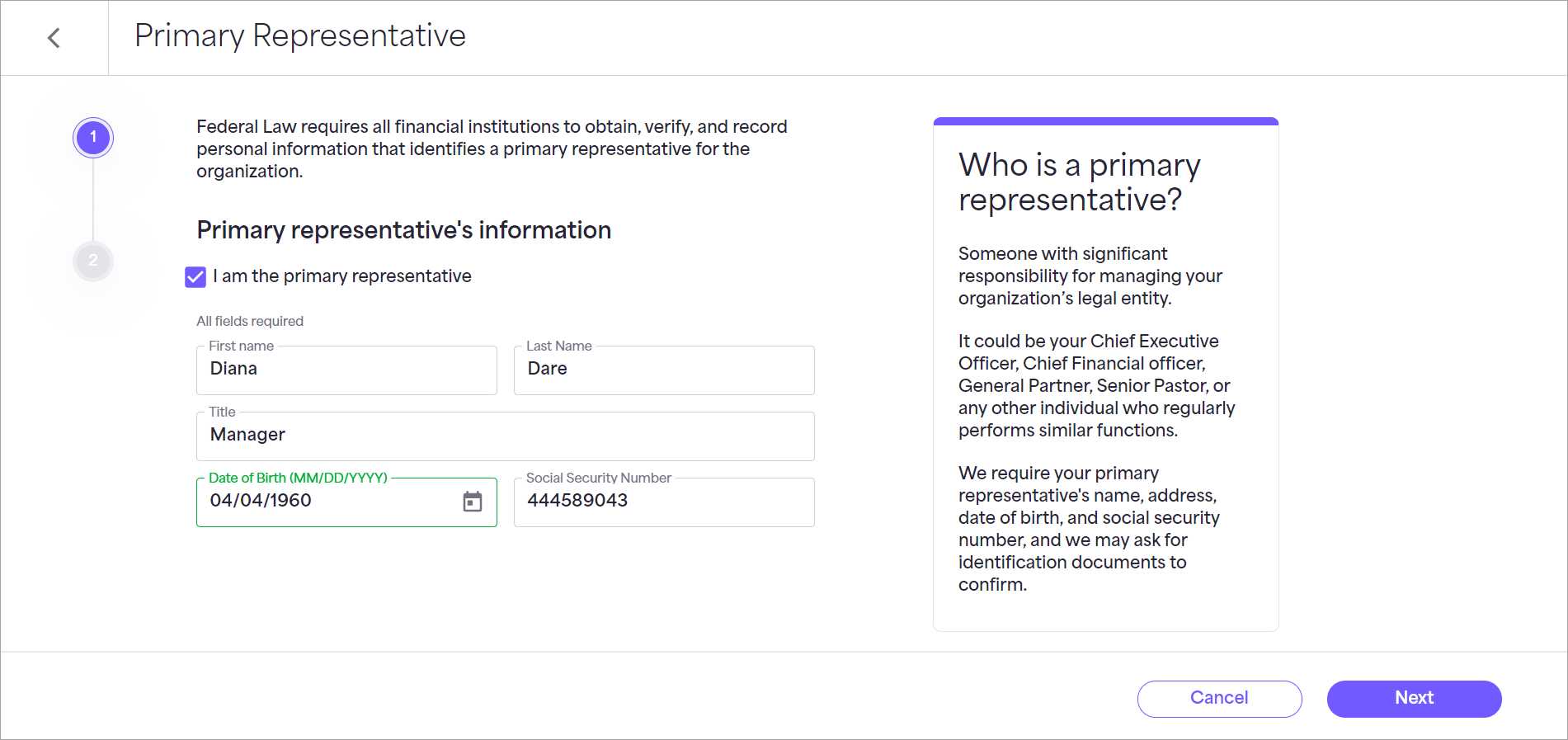The image portrays a webpage titled "Primary Representative." At the top of the page, a notice reads: "Federal law requires all financial institutions to obtain, verify, and record personal information that identifies a primary representative for the organization." Below this notice, there is a section labeled "Primary Representative Information." 

Within this section, a checkbox, highlighted in purple and indicating "I am the primary representative," is checked. An important note follows, stating "All fields required." The form contains the following entered details:

- **First Name:** Diana
- **Last Name:** Dare
- **Title:** Manager
- **Date of Birth:** 04-04-1960
- **Social Security Number:** 589-04-043

To the left, there is a descriptive tab explaining who qualifies as a primary representative. It states that this individual is someone with significant managerial responsibility for the organization's legal entity. This could be a Chief Executive Officer, Chief Financial Officer, General Partner, Senior Pastor, or any other individual who regularly performs similar functions. It details that the primary representative's name, address, date of birth, and social security number are required, and there may be a need for identification documents for confirmation.

At the bottom of the form, there are two buttons: "Cancel" and "Next."